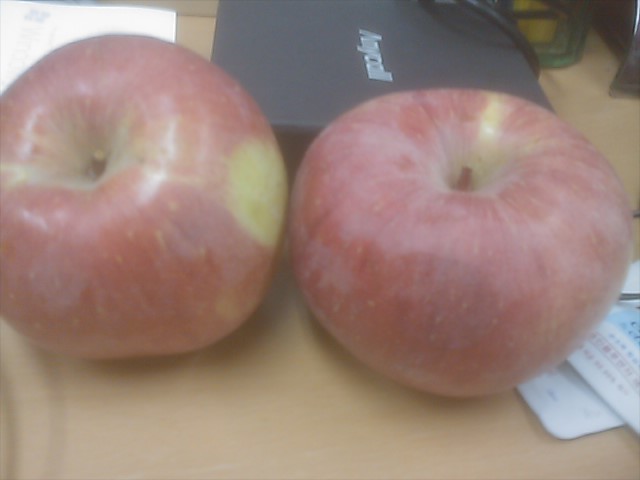The photograph features two apples, most likely Macintosh due to their red and green coloring with a slightly hazy, white finish as if they haven't been washed or polished. These apples sit side by side on a pale beige wooden desk or table, appearing to serve as makeshift paperweights. The left apple anchors a sheet of paper at the upper left corner, while the right apple secures what looks like the ends of boarding passes or tickets in the lower right corner. A black, closed laptop with indistinguishable white text is positioned behind the apples, with green cables emerging from its upper right corner. The image has a slightly blurred quality, giving a soft focus to the apples, while the darker laptop appears slightly sharper in the background.